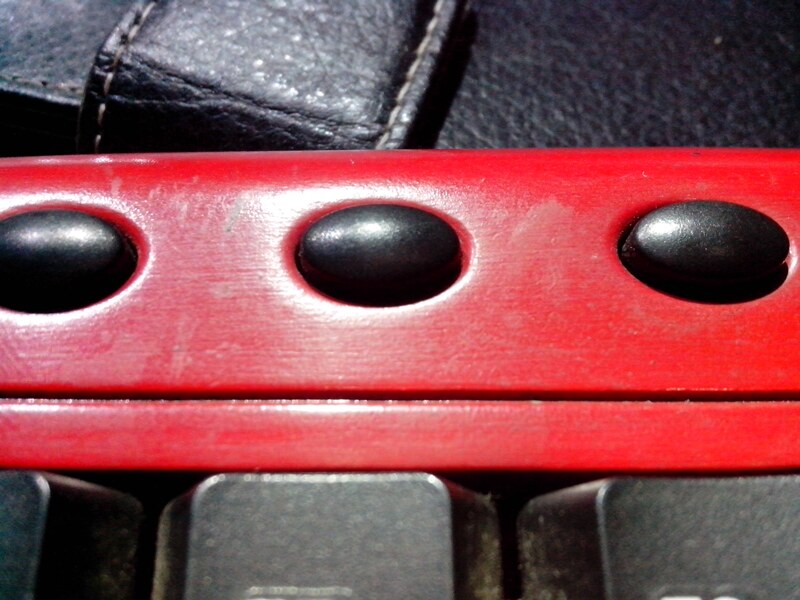This is a detailed close-up photograph capturing a horizontal red metal beam that spans the image from left to right. On this beam are three solid black, horizontally oval-shaped objects. The upper portion of the image showcases a leathery black background featuring a braised leather texture with white stitching along the outer edges. Towards the lower part of the image, there are parts of four rectangular steel platforms, partially visible and resembling cut slabs. The red beam has a polished, shiny surface, suggesting it might be made of a glossy material. While the context is somewhat ambiguous, elements like the black oval shapes and the leather texture hint at possible components of a mechanical or electronic device.